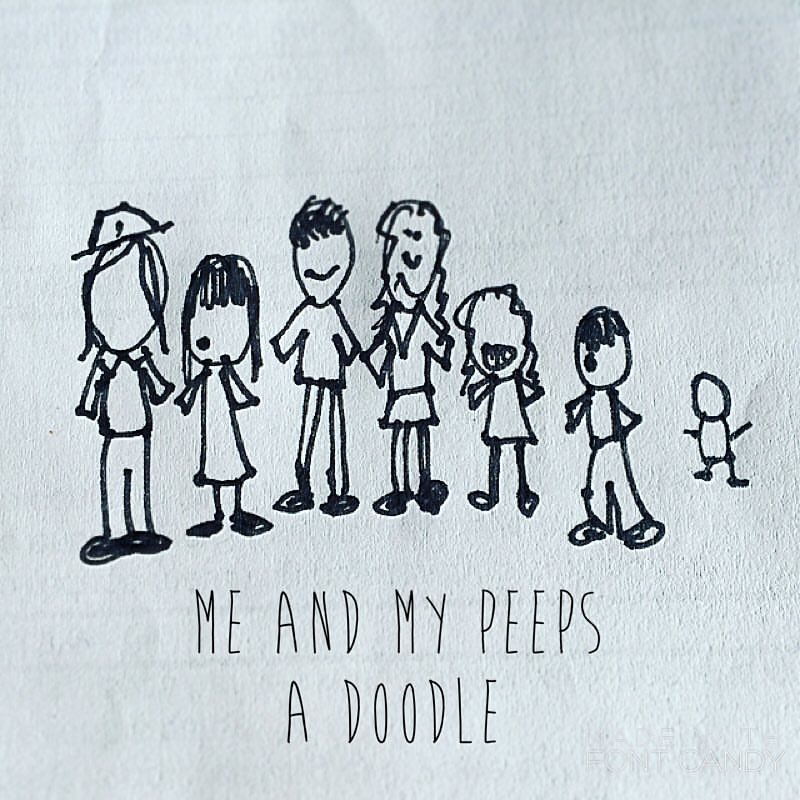This whimsical sketch features a charming array of seven stick figure cartoon characters, each distinguished by unique hairstyles and simple yet distinguishing attire. On the left side of the artwork, four adults are positioned in a row: two women adorned in dresses and two men wearing pants. To their right, two younger children stand, depicted with shorter statures and playful postures. The smallest figure, a tiny baby, is placed furthest on the right, adding a heartwarming touch to the image. Underneath this delightful scene, a handwritten caption reads, "Me and my peeps - a doodle."